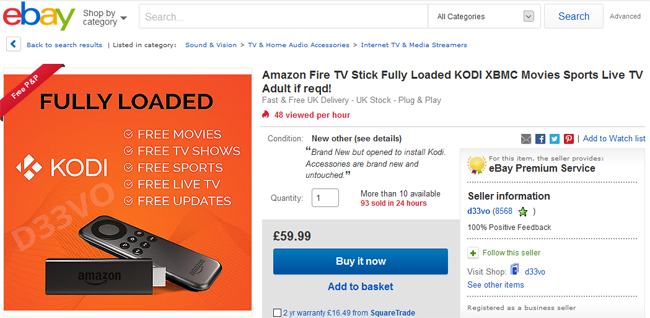This image is a detailed screenshot from a website, specifically eBay. The eBay logo is displayed at the top, with the letters "e" in red, "b" in blue, "a" in yellow, and "y" in green, all in lowercase. Below the logo is a navigation area with a "Shop by category" option accompanied by a drop-down arrow, followed by a search bar. Within the search bar area, there is an "All Categories" drop-down option, a blue "Search" button, and an "Advanced" link.

Below this is a section with navigational aids, starting with a left-pointing arrow within a square, labeled "Back to search results" in blue text. It also indicates the listing's category path in smaller black text: "Sound & Vision > TV & Home Audio Accessories > Internet TV & Media Streamers."

At the top of the main content area, a prominent orange banner reads "FREE P&P." Inside the orange square, bold black capital letters state "FULLY LOADED." The word "KODI" is spelled out in white capital letters, beneath which are promotional phrases: "FREE Movies," "FREE TV Shows," "FREE Sports," "FREE Live TV," and "FREE Updates."

The product being advertised is prominently displayed with an accompanying image of a remote and a streaming stick. The description reads: "Amazon Fire TV Stick Fully Loaded Kodi XBMC Movie Sports Live TV Adult if REQD." It highlights that "40 viewed per hour" and lists the condition as "New Other (see details)." The price is marked at £59.99, and notable labels include "eBay Premium Service" and the seller's information showing "100% positive feedback."

Finally, purchase options are available with "Buy it now" and "Add to basket" buttons.